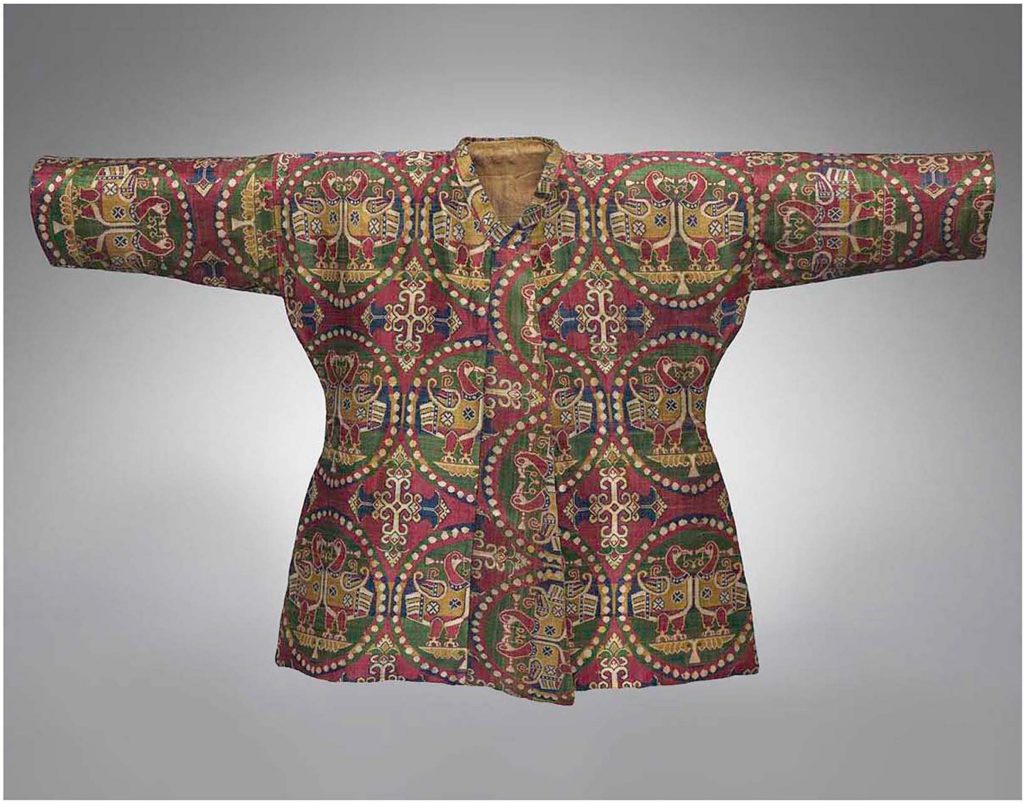In the center of the image, set against a gray background, is a detailed and ornate traditional jacket, appearing to be laid out on a table with its arms spread out straight, giving the impression of standing up. The jacket features three-quarter length sleeves and a small collar. Its dominant color is a faded maroon red, reminiscent of Indian attire. The jacket is closed without buttons and has a tie or fold in the front under the collar.

The fabric displays an intricate and repetitive pattern, predominantly in gold, red, blue, cream, green, and white. Central to the design are pairs of red birds facing each other, seemingly kissing, adorned in golden coats with blue and white emblems that resemble a floral arrangement of four hearts. These birds stand atop golden pedestals, which are encircled by green circles filled with white dots. Surrounding these circles are additional cream circles and ornate crosses, contributing to the jacket's elaborate and ceremonial appearance.